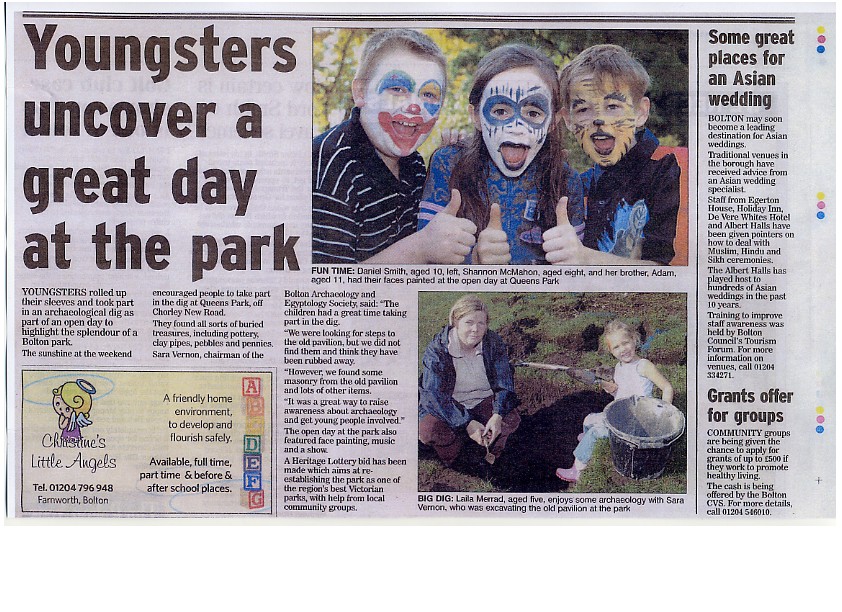The image depicts a newspaper clipping that seems relatively recent, printed on somewhat white paper. The title at the upper left reads, "Youngsters Uncover a Great Day at the Park." The article details how children participated in an archaeological dig to celebrate an open day highlighting the beauty of Bolton Park. On the right, accompanying the text, are pictures of three children with face paint: one as a clown, another as a skeleton, and the third as a lion, all giving a thumbs up. Beneath these images, there is another picture of an adult woman and a child digging a hole with a bucket beside them. In addition, the page includes a lower-left ad for "Christine's Little Angels," and on the right-hand side, there's a column with more news, including sections titled "Some Great Places for an Asian Wedding" and "Grant Offer for Groups." The colors visible throughout the clipping are white, gray, black, blue, red, yellow, orange, green, and purple.